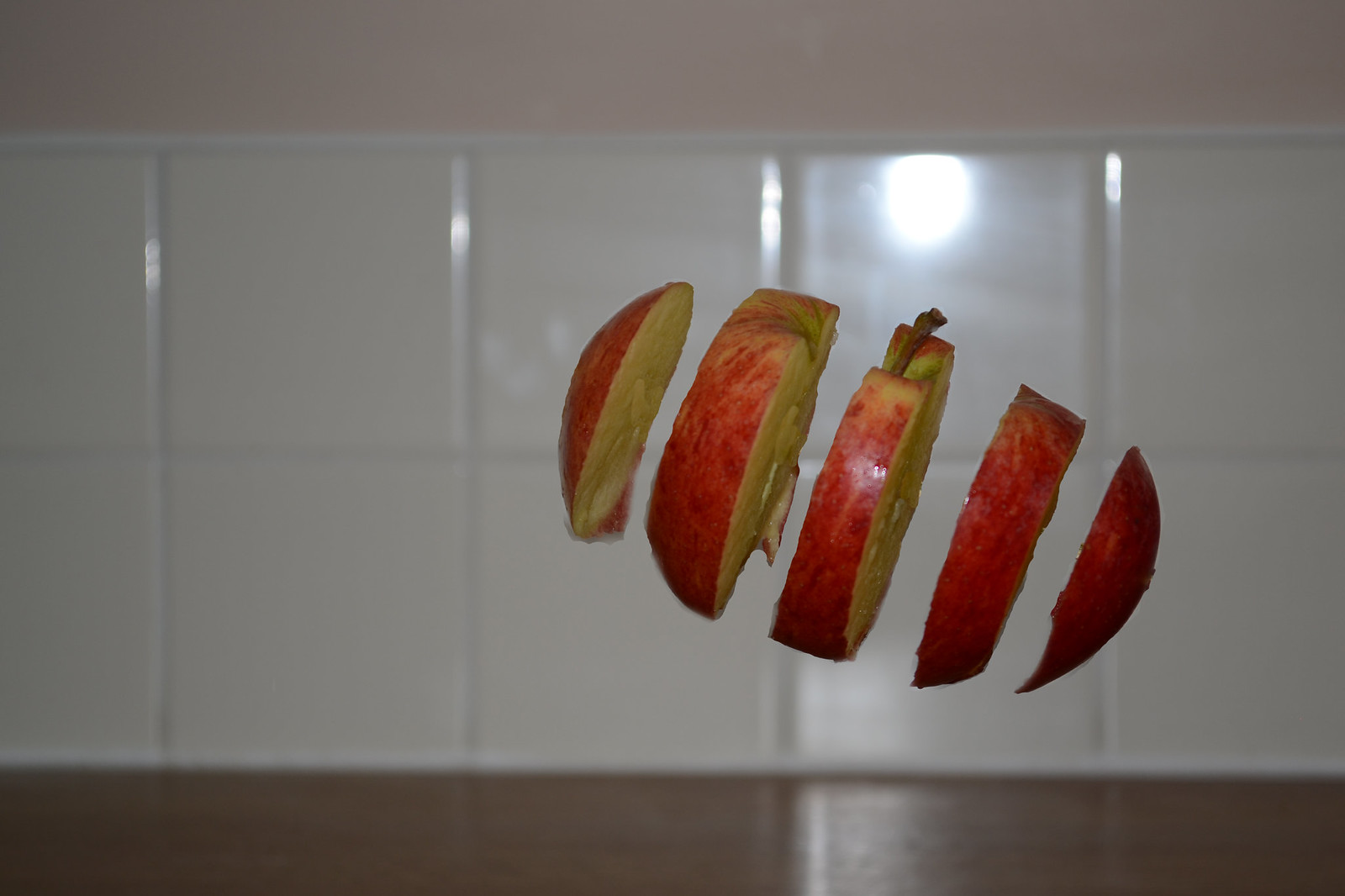This highly detailed photograph depicts a red apple that has been expertly sliced into five sections and appears to be floating mid-air. The apple slices are arranged in a slight leftward tilt, creating an oblong shape with the distinct brown stem visible on the central slice. The interior flesh of the apple ranges from light yellow to slightly oxidized brown, indicating it has been exposed to air for a short while. Behind the apple, the background consists of a polished white tile wall that reflects light, suggesting the use of a camera flash. These tiles, positioned above what appears to be a dark brown or possibly wooden countertop, add a subtle shine. The overall setting seems to emulate a kitchen environment from the 2010s, reminiscent of playful scenes from the Fruit Ninja game. The tiles are square with a slight glossy finish, while above them, a light peachy wall color adds warmth to the composition. The combined elements give the image a realistic yet almost digitally created look, enhancing the impression that the apple slices are suspended in mid-air, possibly with some hidden support or post-editing techniques.